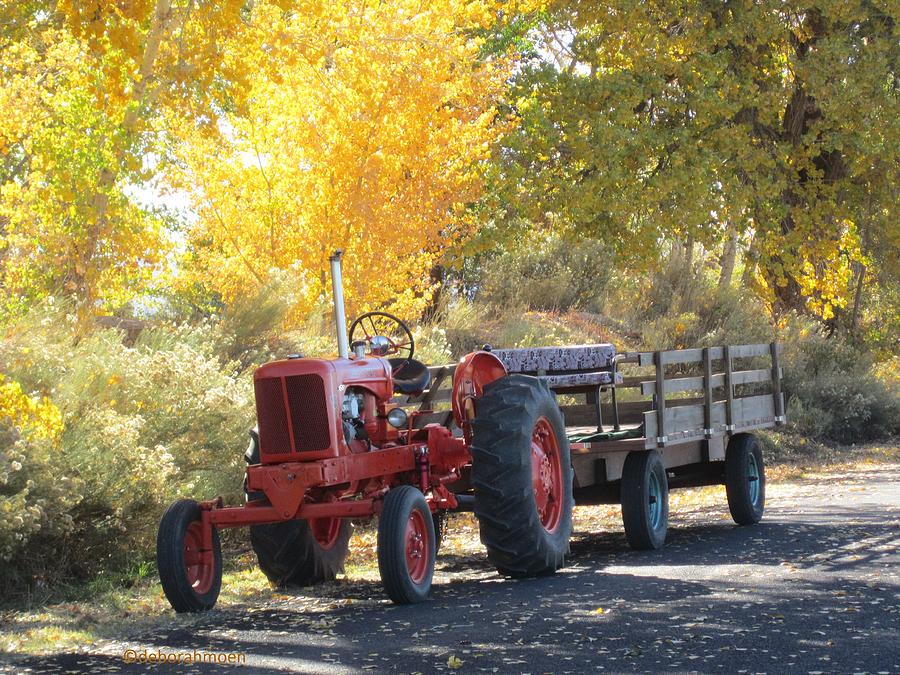A red metal tractor with large black wheels is stationary on a small paved path, pulling a wooden trailer typically used for hayrides, complete with a bench. The scene is set on an autumn day, with the surrounding foliage displaying a vibrant tapestry of colors. To the left, trees with brilliant yellow leaves are illuminated by sunlight filtering through the branches, while another tree behind the tractor shows a mix of green and early yellow leaves. Adjacent to the tractor is a variety of shrubbery, exhibiting a spectrum of yellow, tan, and green hues. Shadows of the trees stretch across the path, adding depth to the idyllic autumn setting. In the bottom left corner, the image is credited to Deborah Moen, with the text in highlighted brown and yellow-orange tones. The narrow path extends from the bottom left corner towards the right, framing the rustic charm of the parked tractor and its wooden load.